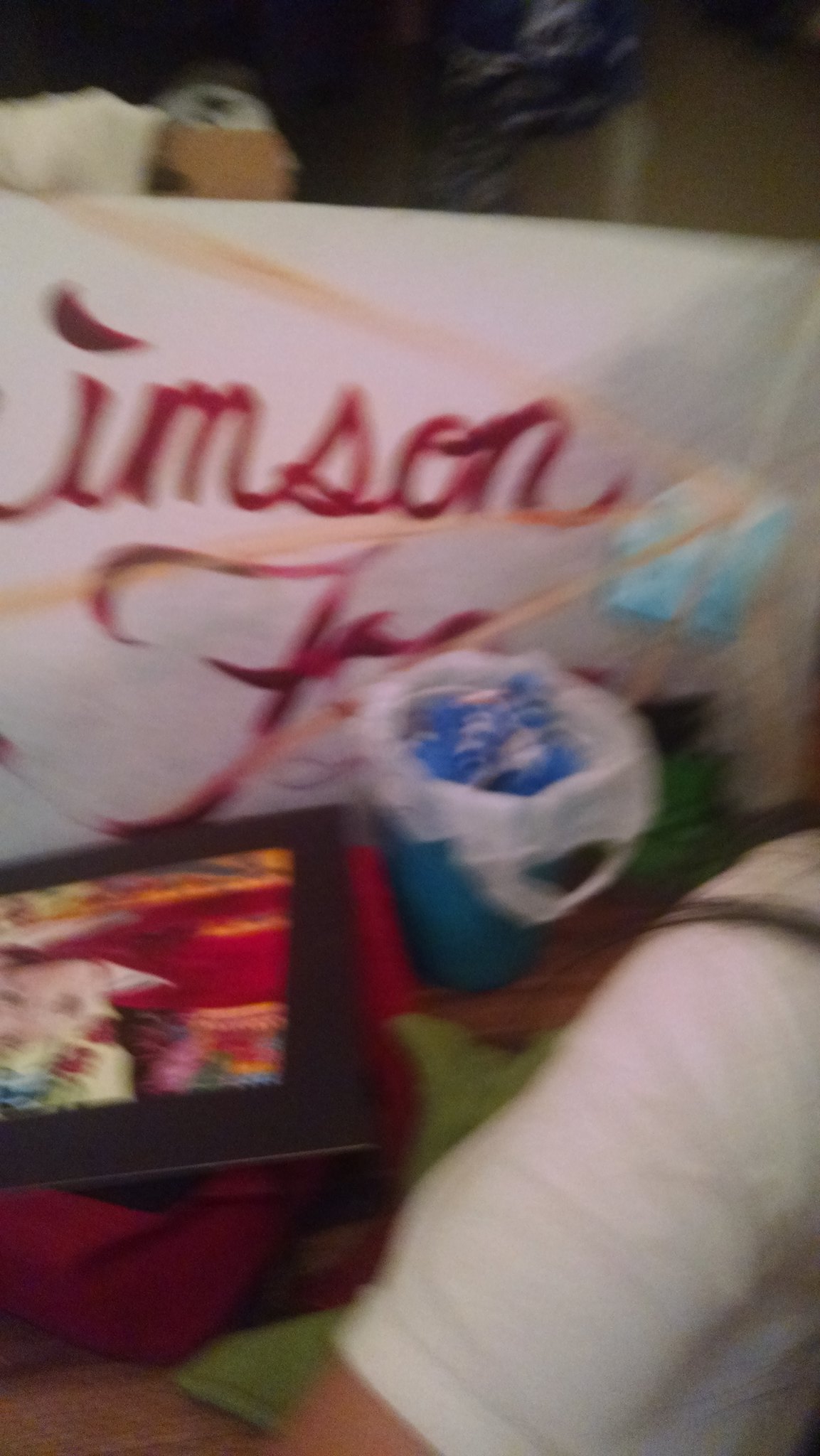In the photograph, a person, identifiable by their shoulder, arm, and part of their chest, is seen passing through a cluttered room. The individual, who appears to be Caucasian, is wearing a white, medium-sleeve shirt and occupies the bottom right quadrant of the image. Behind them, partially obscured, is a white poster with red cursive text that reads "I am S-O-N" followed by an "F" and additional text hidden by other objects. A blue bucket containing a white trash bag and various blue items also obscures the poster. Additionally, there is a drawing of a blue cube with golden lines emanating from it. The room is further detailed by the presence of a red backpack and a black-framed picture of a dog, adding to the miscellaneous array of objects in the scene.